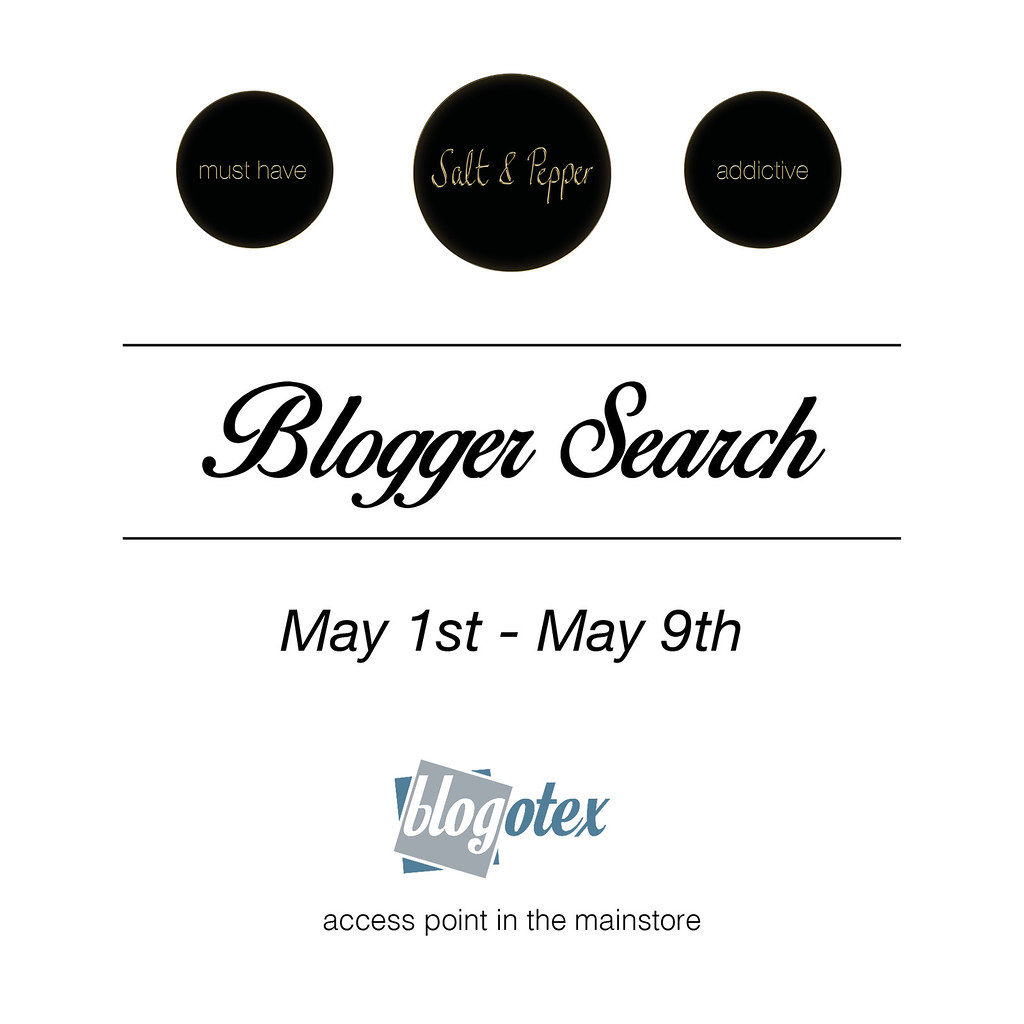The image is a detailed black and white infographic with a clean, minimalist design. It has a portrait orientation and features a white background that blends seamlessly into the edges of the interface. At the top of the image, aligned in a horizontal row, are three black circles with gold text inside. The text in the circles reads "Must Have," "Salt and Pepper," and "Addictive" from left to right. 

In the center of the image, there's a prominent heading in black script font that reads "Blogger Search," flanked by thin black lines above and below it. Beneath this heading, the text "May 1st to May 9th" is written in black italic font. 

At the bottom of the image, there is a logo with the word "Blogotex." The word "blog" is displayed in white script against a gray square set on a diagonal, overlaid on a blue square, while "otex" is in blue script. Below this, in black text, it says "Access Point in the Main Store."

The overall design suggests it could be an advertisement or something typically seen on a website, emphasizing clean and modern infographic typography.